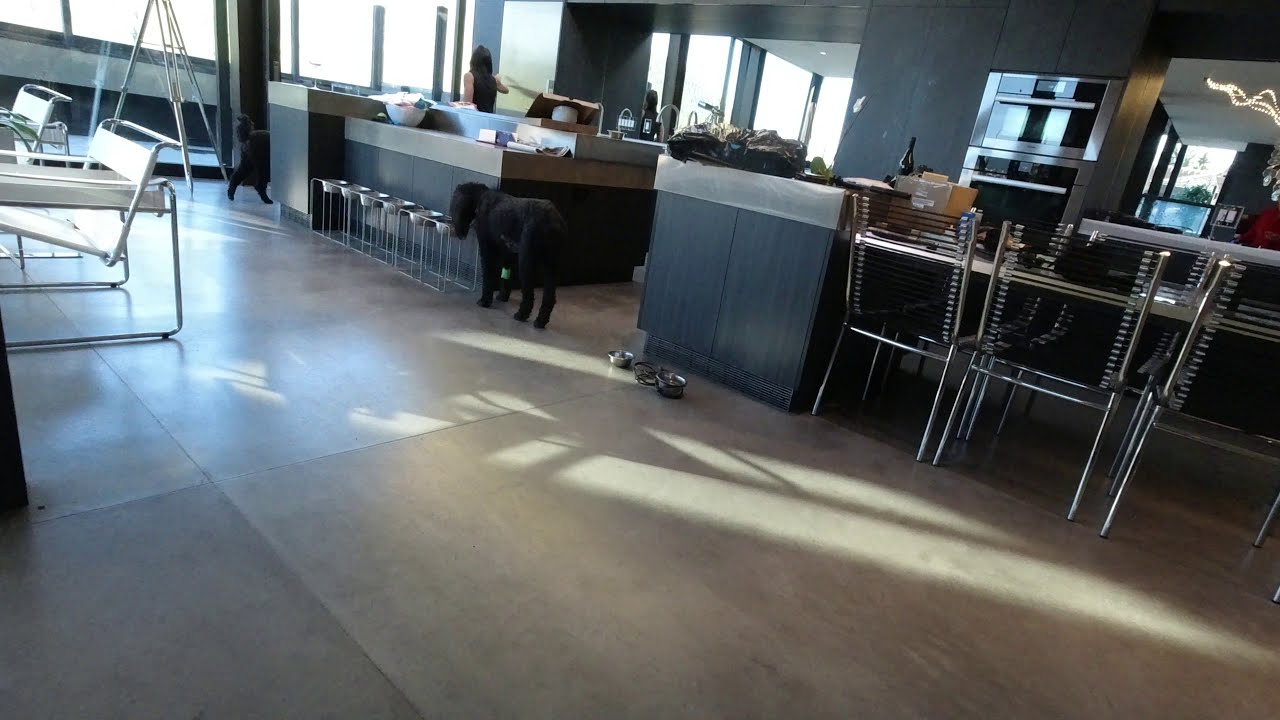The detailed caption for the image could be:

This bright, indoor daytime photo captures a sleek, modern kitchen, primarily decorated in dark gray tones with integrated stainless steel and black appliances. The stylish countertops, possibly made of marble or granite, are gray and cluttered with an assortment of bowls, boxes, plastic bags, and garbage bags. The focal point of the kitchen includes a gray counter with a matching table area, beneath which are uncomfortable, steel-rodded chairs and several stainless steel stools, likely part of a breakfast bar setup.

In the kitchen's center are two tall, black dogs. One stands near a row of elevated dog bowls, appearing to drink, while the other enters the kitchen area, close to a woman who has long brown hair and is wearing a dark sleeveless top. She stands on the left side, gazing out a window that allows ample daylight to flood in. The space is characterized by a brownish cement floor composed of large, cornered blocks. 

Further decor includes black and metal kitchen chairs around a kitchen table and stainless steel and white chairs resembling lawn loungers. The overall ambiance suggests a place where design is prioritized, hinting at a meticulously curated but perhaps less comfort-focused aesthetic.